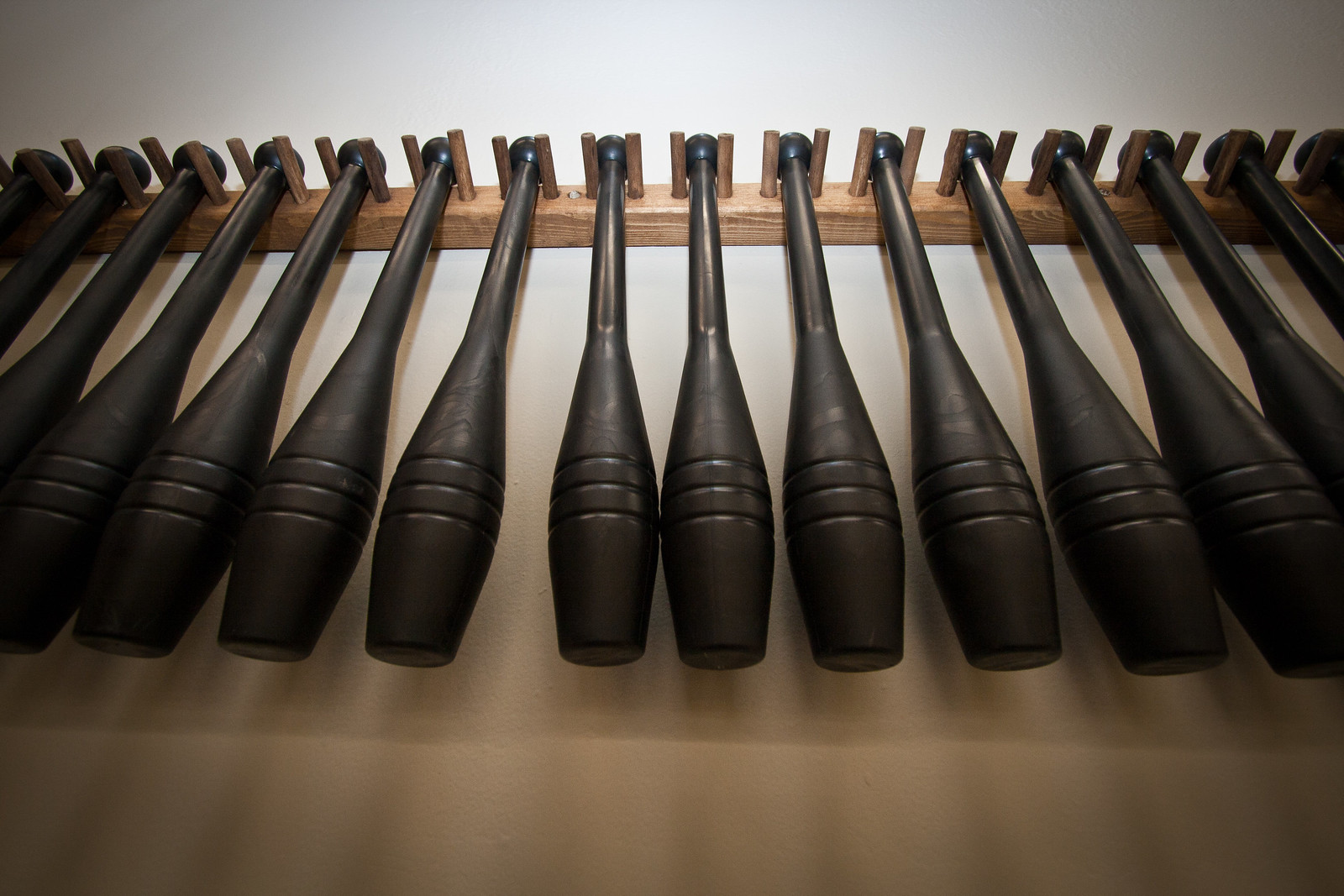In this rectangular, color photograph, we see a collection of approximately 16 identical black objects hanging from a long, light brown wooden rack mounted on a white wall. The photo was taken indoors from a slightly lower angle, looking up the wall. Each object resembles an elongated bowling pin or an antique baseball bat, characterized by a flared, wide bottom and a thinner, cylindrical handle.

These objects, likely made from a heavy material such as plastic or wood, feature three equidistant grooved rings near the wider part of the form. They're suspended by the handles on short dowels that protrude from the rack. Shadows of the bats are cast sharply on the wall beneath them. The rack appears to be constructed from natural, unfinished pine and is bolted securely to the wall. The overall appearance of the scene suggests careful organization and a sense of geometric uniformity.